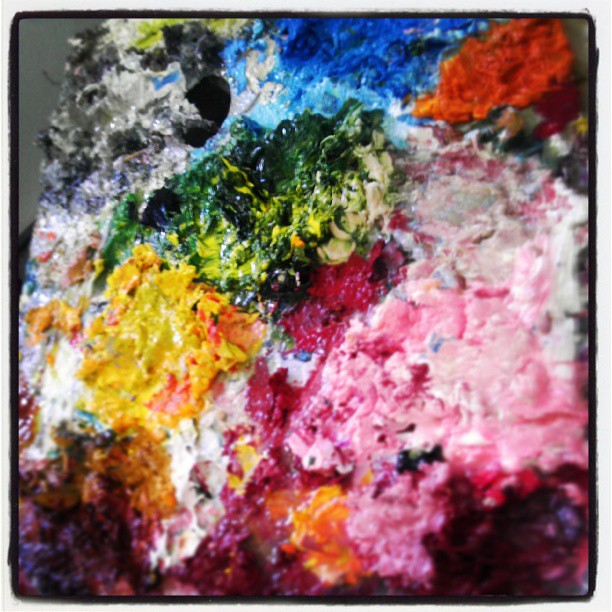The image showcases a highly textured and vibrant art piece, possibly a close-up of a painting or palette, with an impressive array of colors scattered throughout. Dominating the center is a dark green area, surrounded by yellow and topped with a gradient of blue, transitioning from a lighter to a darker shade. To the right of the blue, there's a very dark orange hue that stands out. The lower left corner is marked by dark pink or purple tones, while the top left features a gray shade. The right half of the image prominently displays shades of white, light pink, and dark pink. The entire composition is highly textured, resembling the thick and uneven application like that of oil pastels. The paint appears almost wet and shiny, emphasizing the three-dimensional quality of the piece. The chaotic blend of colors and textures creates a dynamic visual experience, suggesting it could also be a photograph of a human-painted, multicolored rock formation, with jagged surfaces and a distinct black frame enveloping the whole scene.